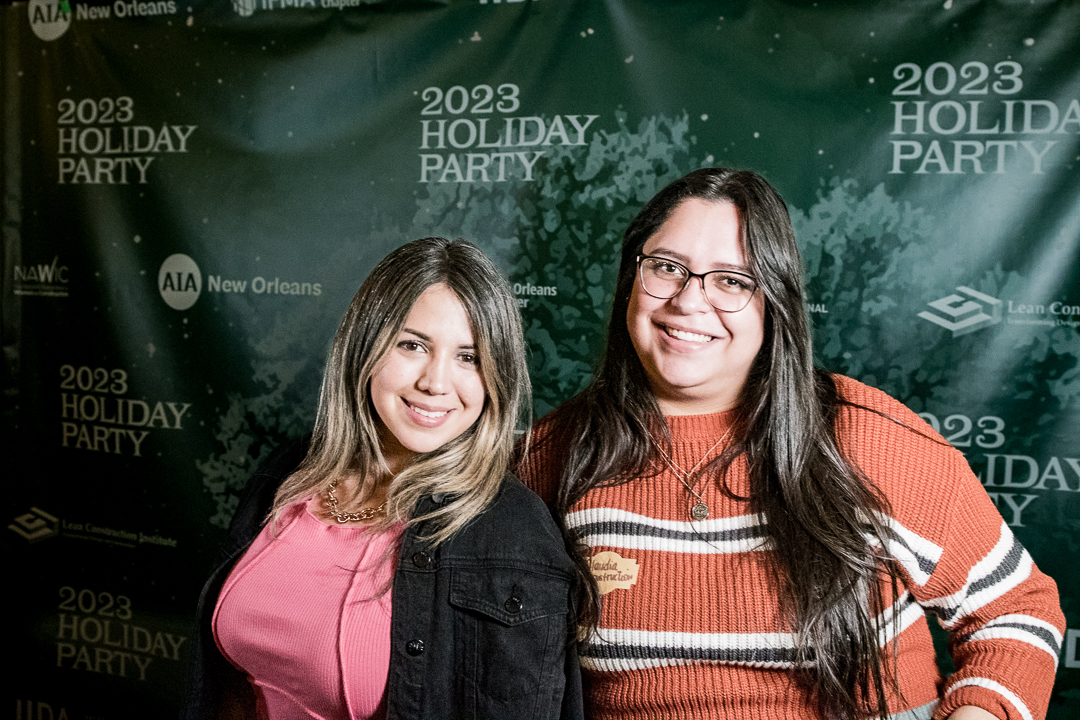In the photograph, two women are standing close together, smiling as they pose for the camera. The backdrop features a large, dark green canvas banner, adorned with scattered white specks and artistic images of trees in various shades of green. Across the top, in prominent white letters, the text "2023 Holiday Party" is repeated, accompanied by logos of sponsors, including AIA New Orleans, though the other logos are not clearly visible due to the blurriness of the background.

The woman on the left has long, lighter brown hair and is dressed in a dark jean jacket over a pink shirt, accessorized with a gold necklace. The woman on the right, with darker brown hair, is wearing glasses, an orange sweater with white and black stripes, and is smiling warmly. The photograph appears to have been taken indoors using a flash, highlighting the subjects against the dimly lit festive backdrop.